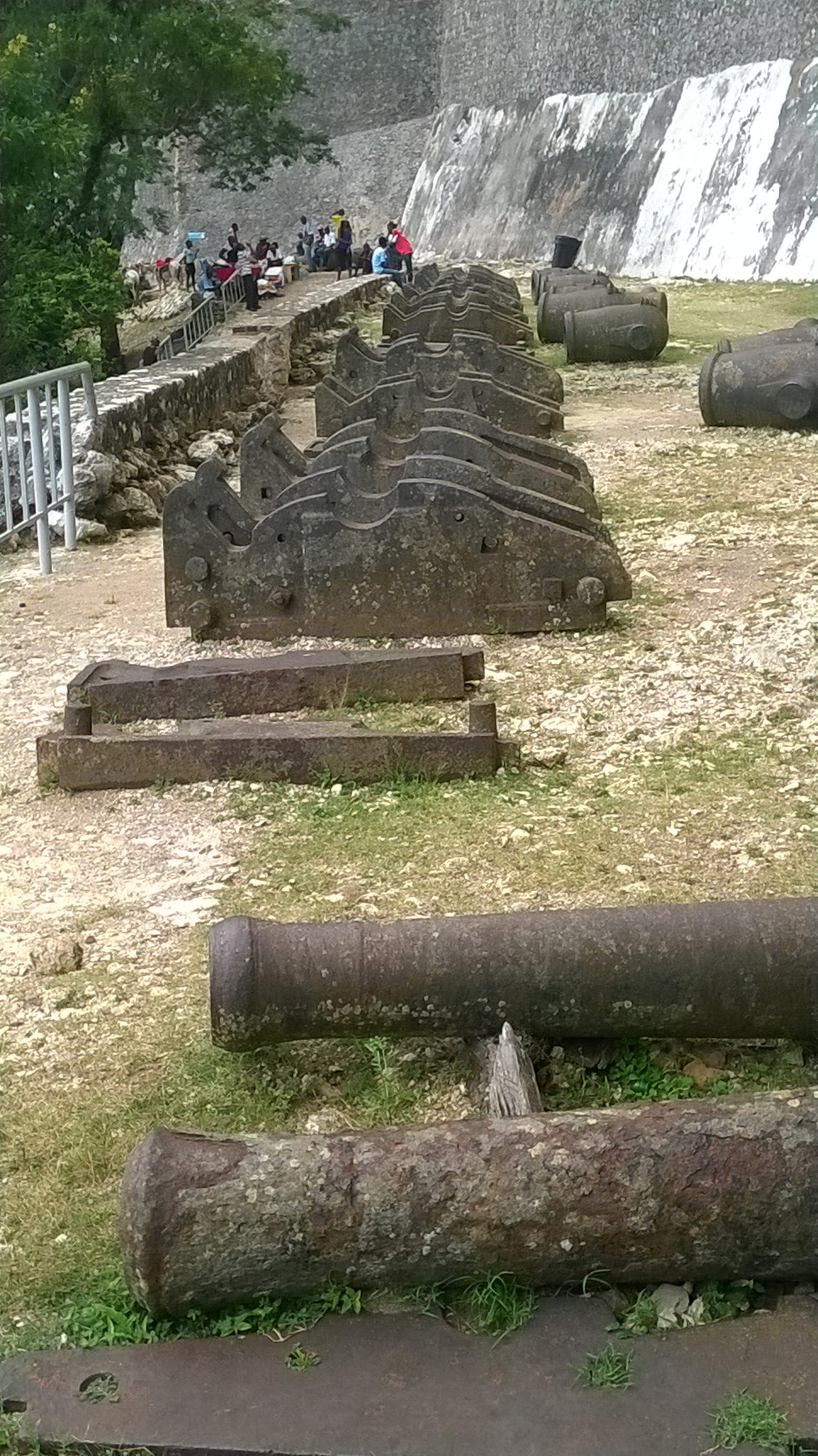This detailed outdoor photograph captures a historical fort, with several noteworthy elements. In the foreground, two rusty metal cannons lie on a patch of dead or matted grass, framed by two long, ambiguous objects that might be wood or metal. Proceeding into the background, there is a neat row of about a dozen old cannon carriages or holders without the cannons themselves. Interspersed amongst them are several large, rusty pieces of machinery or metal parts, echoing the fort's antiquated ambiance. To the left, a silver handrail accompanies a stone wall, and trees partially obscure the fort's gray, weighty stone walls. The rocky walkway in front of the fort is scattered with visitors, the colors of their clothes—red, blue, black—standing out against the scene's earthy tones. The entire display rests on a dirt or grass surface, capturing the juxtaposition of historical relics and natural elements in this picturesque setting.